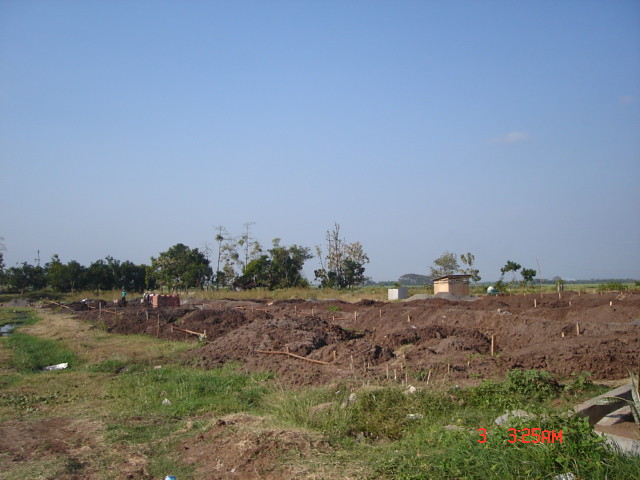The image captures an outdoor setting during a clear, daytime sky with a lone grayish-white cloud drifting in the middle of the otherwise blue expanse. In the distant background, there are trees and small shacks or buildings. The central focus of the image is a green field that has been extensively dug up, resulting in numerous mounds of dirt scattered across it. The field features wooden sticks connected by string, suggesting a rudimentary layout or marking of plot boundaries. Patches of grass are visible amidst the dirt piles. The bottom right corner of the image displays text reading "3" and "3.25 AM."